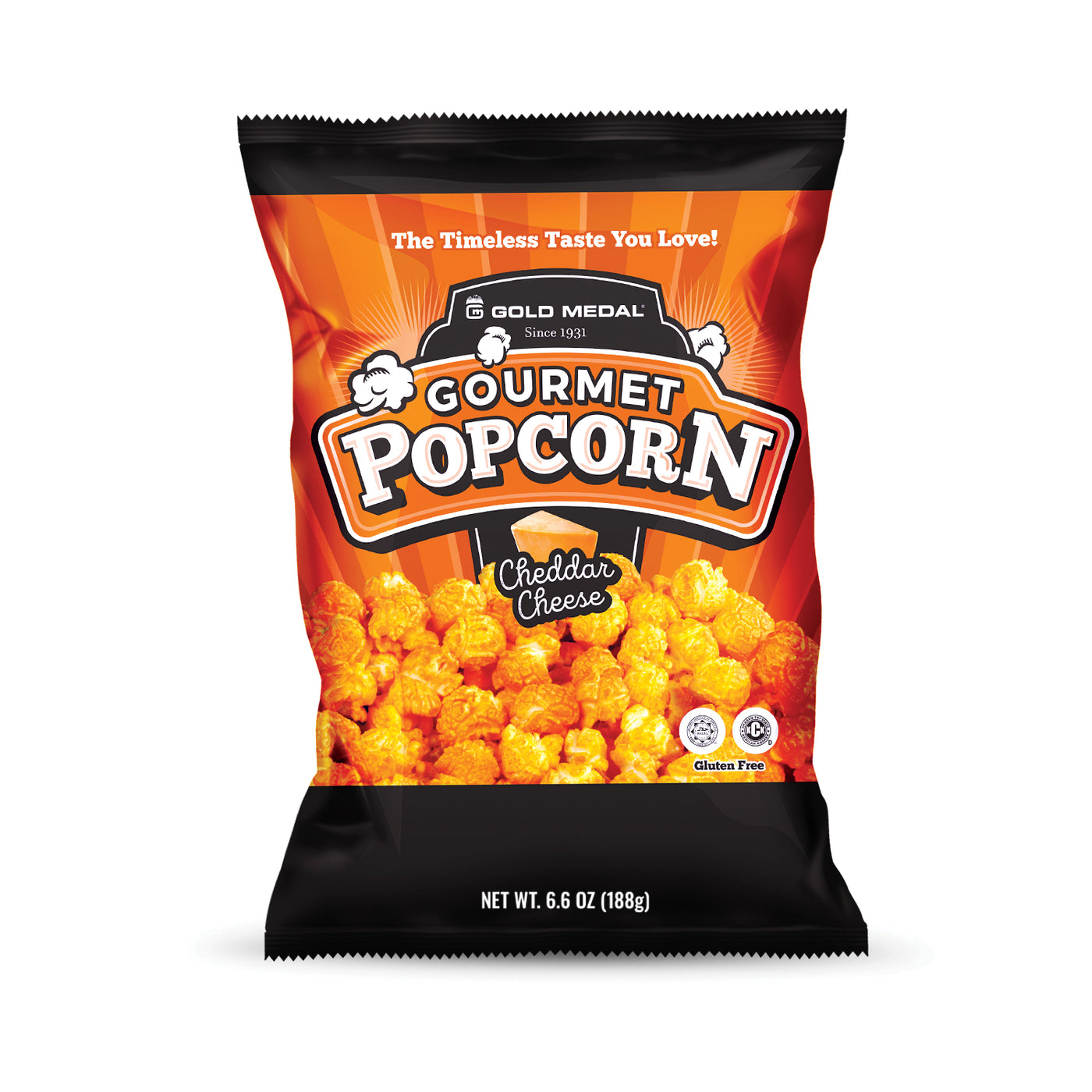The image showcases a gourmet popcorn bag by Gold Medal, prominently featuring the slogan "The timeless taste you love." The packaging is visually striking with a combination of black, orange, gold, and cream colors. At the top, the bag displays the phrase "Gold Medal since 1931" in white letters on a black background. Below, "gourmet popcorn" is boldly written in white with a black outline against an orange background. The flavor, "cheddar cheese," is highlighted on a small black banner. The bag showcases an appetizing picture of orange and yellow cheddar cheese popcorn across the center and bottom portions. The bottom-right corner includes labels indicating the product is gluten-free and weighs 6.6 ounces (188 grams). The bag also features Hebrew writing, suggesting the product may be kosher. White kernels and a wedge of cheddar cheese further accentuate the attractive design, making it visually appealing and informative.